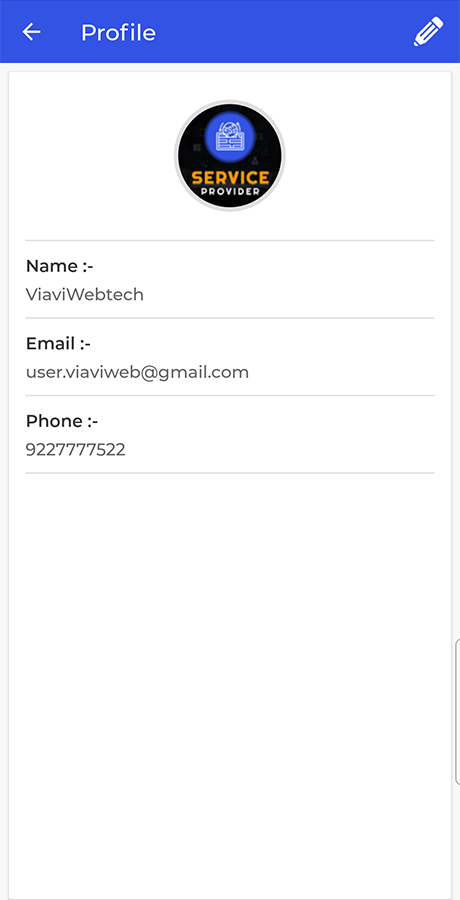The image features a user interface with a blue header at the top. On the left side of the header, there is a white arrow pointing left, labeled "Profile". On the right side, a pencil icon is displayed. 

Directly below the blue header is a gray-outlined rectangle. At the top of this rectangle is a black circle with a gray outline, containing a blue circle inside it, which resembles an open book with a smaller circle on top. The text within the rectangle reads "Service" in orange and "Provider" in white.

Beneath these labels, a gray line separates the header from the following user details section:
1. **Name:** "BIABIWEBTECH", marked with a colon.
2. **Email:** "User.B-Web@G-Mail.com", marked with a colon.
3. **Phone:** "922-777-522", marked with a colon.

Each of these sections is separated by gray lines. The area beneath the phone number section is blank.